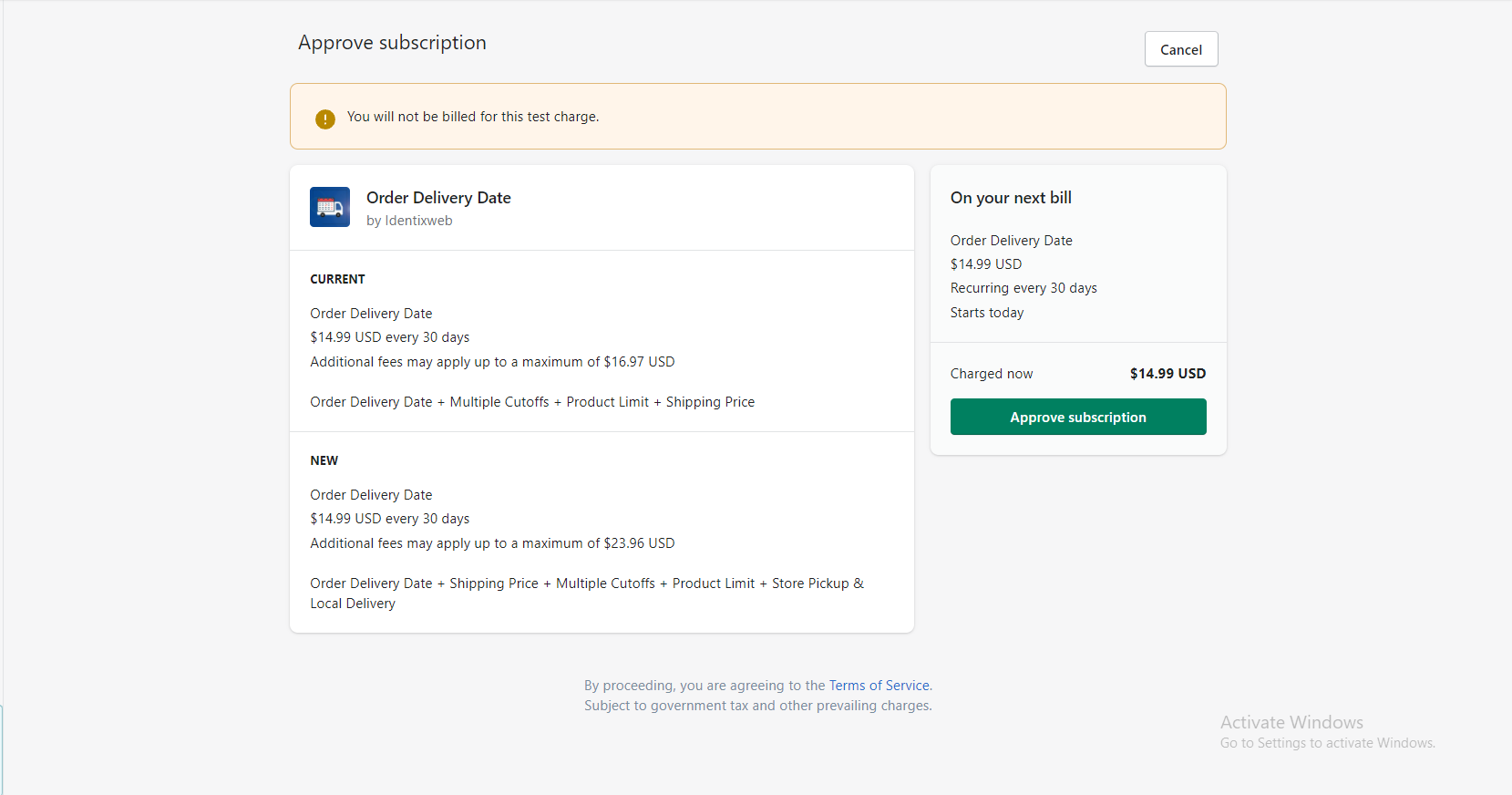In the image, a grey-background webpage is displayed. At the top left, the text "Approve Subscription" is prominently featured. Positioned at the top right is a white button labeled "Cancel." Just beneath these elements, there is a brown-background section with the text "You will not be billed for this test charge." 

To the left side, there is explanatory text starting with "Order delivery date by Identix Web," accompanied by a blue-background icon of a truck in delivery motion. Below the icon, the text outlines the current order details: "Current Order Delivery Date: $14.99 USD every 30 days. Additional fees may apply up to a maximum of $16.97 USD. Order delivery date plus multiple car ops plus product limits plus shipping price."

Further down, a new set of order details is featured, starting with "New." Here it's noted: "Order delivery date: $14.99 USD every 30 days. Additional fees may apply up to a maximum of $23.96 USD. Order delivery date plus shipping price plus multiple car ops plus product limits plus door pickup and local delivery."

On the right side, a message indicates the billing details: "On your next bill, order delivery date: $14.99 USD recurring every 30 days, starts today, charge now," with the price prominently displayed as $14.99 USD. Below this, a green button prompts the user with "Approve Subscription."

At the bottom of the page, outside the main text areas, there is a disclaimer: "By proceeding, you are agreeing to the terms of service subject to government tax and other prevailing charges." In the bottom right corner, a system alert is shown reading "Activate Windows, go to Settings to activate Windows."